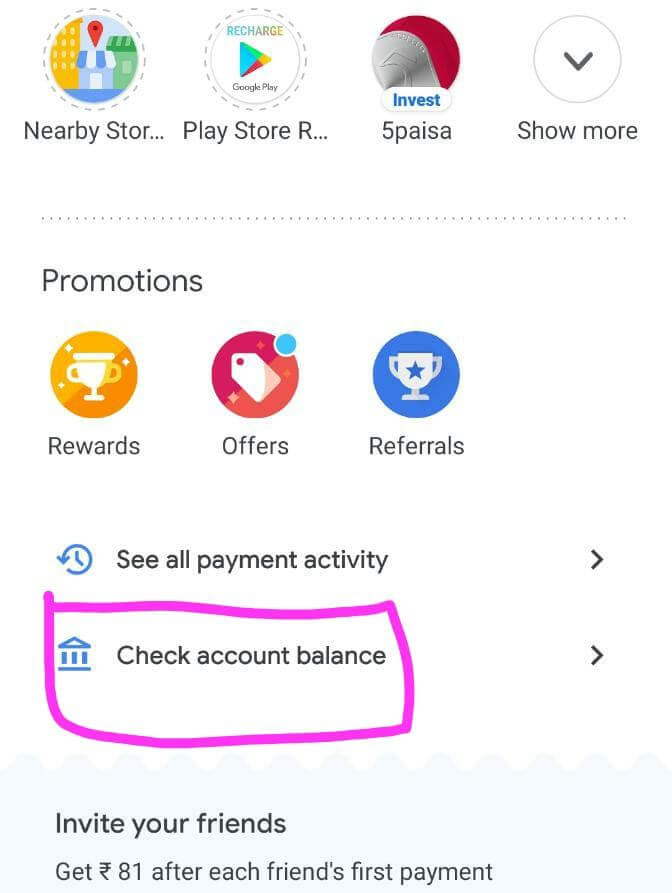This image appears to be a screen grab from a financial application. Displayed on a white background, the first row features four circles, each representing different functionalities:

1. **Nearby Store**: Depicted in a blue circle featuring a gold, blue, and green building icon, with a red pin over it.
2. **Recharge Google Play**: Shown in a white circle with a green, burgundy, and gold play button icon. The text partially reads "Google Play Store," though it is truncated.
3. **Blue Invest - 5 Paisa**: Enclosed in a red and silver circle with the company name displayed prominently.
4. **Show More**: Represented by a white circle with a gray arrow.

The second row of circles includes:

1. **Promotions**: A gold circle with a white cup icon labeled "Rewards."
2. **Offers**: An orange and pink circle with a white price tag icon.
3. **Referrals**: A blue circle featuring a white trophy with a blue star, labeled "Referrals."

Below these rows, additional functionalities are outlined:

- **Payment Activity**: Illustrated by a blue clock icon, a black "CL Payment Activity" label, and an adjacent arrow.
- **Check Account Balance**: Indicated by a blue icon resembling columns, a black label "Check Account Balance," and a pink square around the text.
- **Invite Friends**: Detailed at the bottom, the black text reads, "Invite your friends, get £81 after each friend's first payment," accompanied by an arrow.

Overall, the image effectively displays various features and promotions available within the financial application.